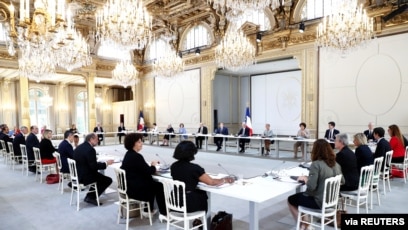This horizontally aligned, smaller-sized rectangular image showcases a group of approximately 30 to 40 individuals gathered in a large, opulent conference room for what appears to be an official meeting, likely involving legislative or policy discussions. The attendees are seated in white chairs around a substantial, U-shaped white wooden table that dominates the room. The table, designed to facilitate face-to-face interaction, has a large rectangular cutout in the center, possibly intended for speakers, though currently unoccupied. The people, mostly dressed in black or gray attire, with one woman in red standing out on the right side, each have microphones in front of them on the table.

The room exudes grandeur with its gold-colored walls adorned by distinctive beige square panels featuring circular designs at their centers. Behind the attendees, horizontal stripes of blue, white, and red flags punctuate the setting. Adding to the room's luxurious ambiance are at least eight magnificent chandeliers, beautifully lit and hanging from the tall ceilings. The bottom right corner bears the "Via Reuters" watermark, indicating the source of the image.